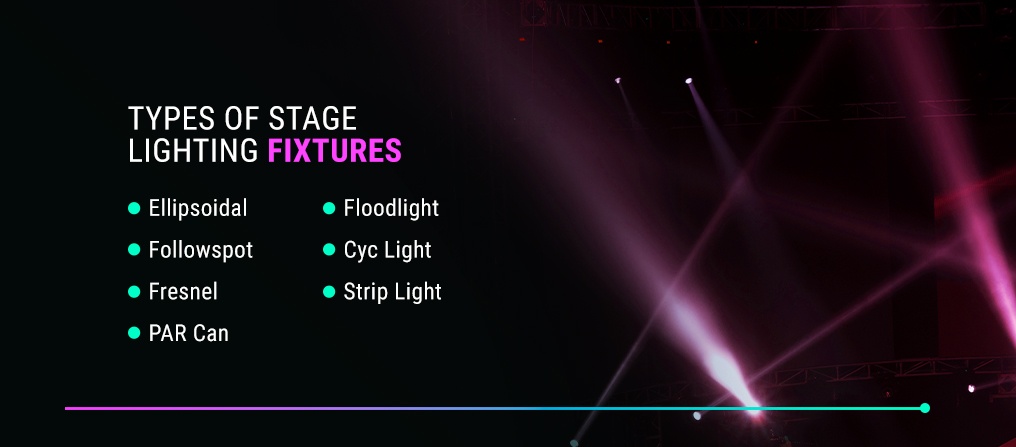This graphic-generated infographic focuses on various types of stage lighting fixtures, set against a largely black background. On the left side, white text prominently lists different types of stage lighting: Ellipsoidal, Follow Spot, Fresnel, PAR, Floodlight, CYC Light, and Strip Light, under the title "Types of Stage Lighting Fixtures." The word "fixtures" is distinguished in a pink or purple hue. At the bottom of the image, a gradient bar transitions from hot pink to purple and then to aqua. On the right side, beams of light, primarily pinkish, purplish, and white, emanate from the lower right corner, representing spotlights and dispersing upward and to the left. The design suggests an educational purpose, typical of content found in web pages or books explaining stage lighting equipment.